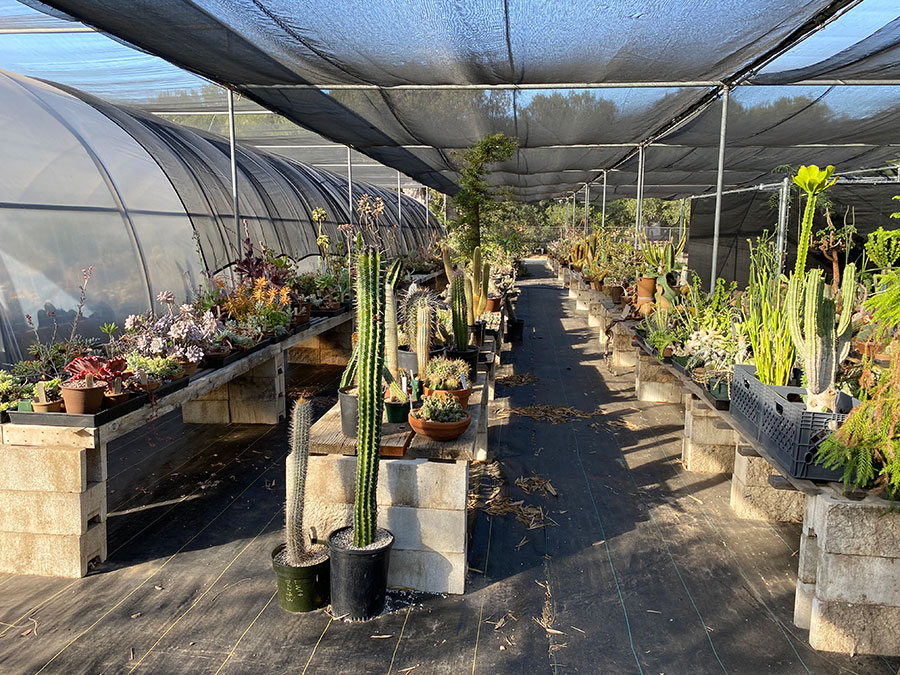The photograph captures the interior of a muted-colored greenhouse, predominantly filled with various cacti and succulents arranged in pots. The greenhouse features a wooden floor, with wooden shelves supported by cinder blocks extending in two aisles that lead the view deeper into the space. A defining feature is the roof, covered by a black mesh material held together with metal tubing and bars, which filters the bright sunlight, casting intricate shadows on the plants below. To the left, there is a separate, round-topped greenhouse structure also covered in mesh. The plants themselves vary in size and color; bright green hues—enhanced by the sunlight—gradually transition to softer, muted tones where the light is diffused by the mesh. The arrangement includes three rows of plants, with the middle row showcasing orange flowers, surrounded by tall, singular cacti and smaller grey cacti lined on the left. The overall scene is a tranquil display of organized botanical diversity, set against a backdrop of natural light and structural elements.